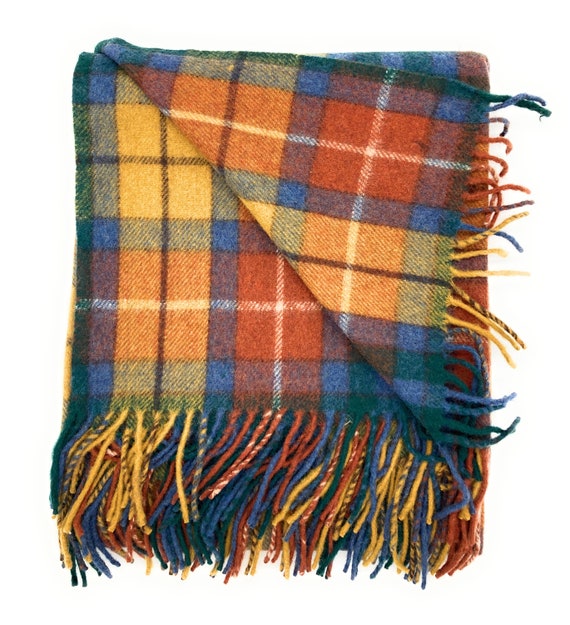This image portrays a cozy, folded plaid throw blanket or large scarf, likely made of wool, resting on a white background. The tiny plaid pattern showcases an array of colors: green, blue, yellow, orange, red, and hints of a purple hue. One corner of the blanket is folded over, creating a triangular section that reveals both the inside and outside of the fabric. The edges are adorned with a long, curly twisted fringe composed of intertwining threads of matching colors, including combinations like yellow and blue, yellow and gray, and red and white. The blanket's fuzzy texture and vibrant, interwoven design make it visually appealing and inviting.